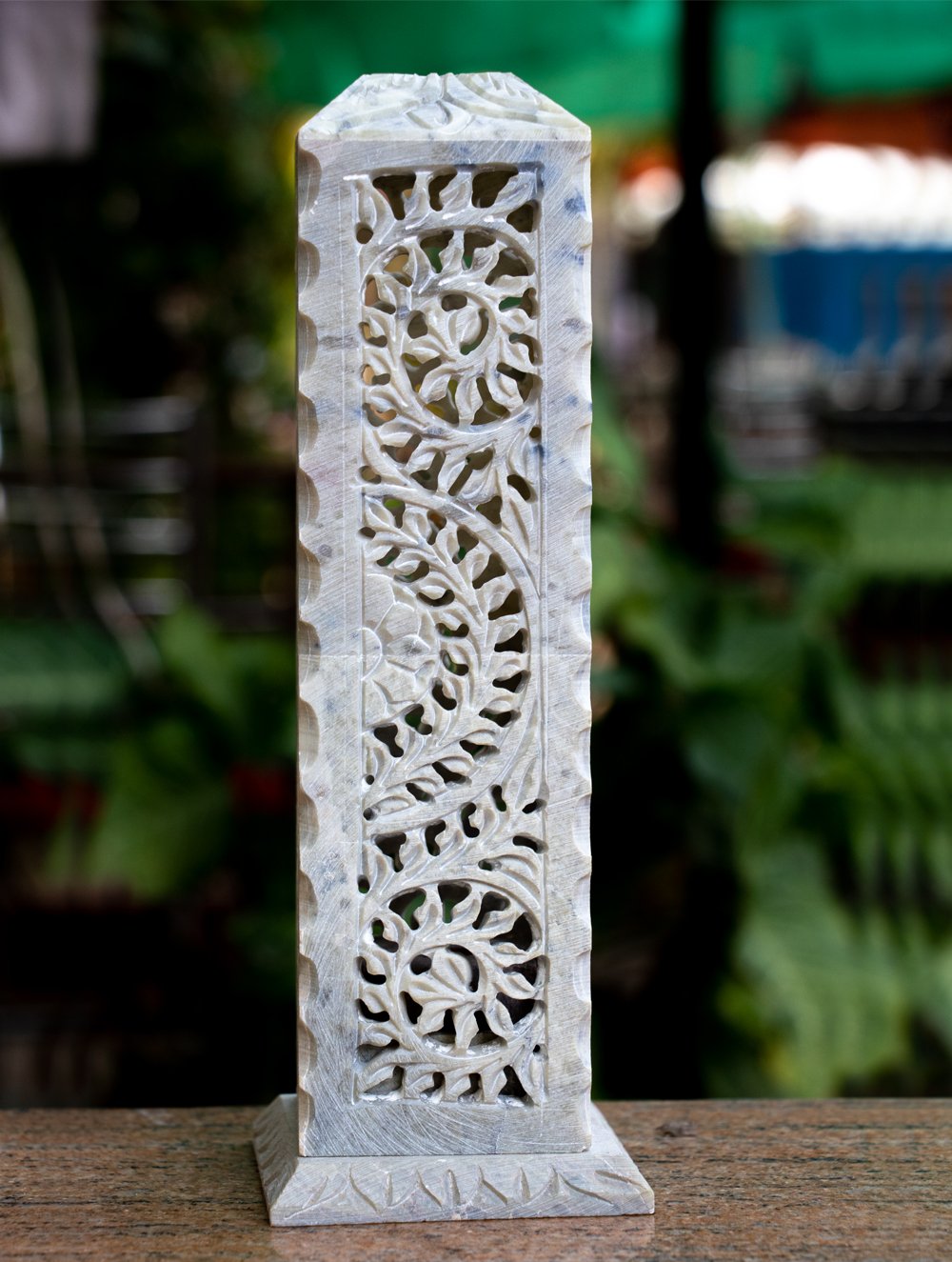The image showcases a detailed, stone-like figurine resembling a small tower or temple, approximately two to three feet tall, placed on a brown wooden table with gray specks and occasional blue dots. The figurine, made from a hard, gray substance, features a rectangular structure with a base adorned with leaf carvings. It has intricate spiral patterns, flower motifs, and vines etched into its surface, which pierce through the material, creating see-through sections. The background is blurred, but hints at green-colored chairs and some lights and vegetation, adding a subtle, out-of-focus ambiance to the scene.